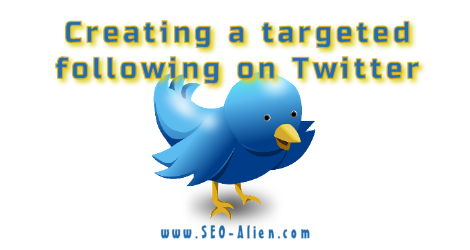A blue-feathered bird with a yellow beak and yellow feet is the centerpiece of the image, prominently engaging in building a targeted following on Twitter. The text in the image reads "creating a targeted following on Twitter," and the image features a yellow border with a white background that casts soft shadows beneath the bird. The website "www.seo-alien.com" is displayed multiple times, reinforcing the theme of strategic social media growth.